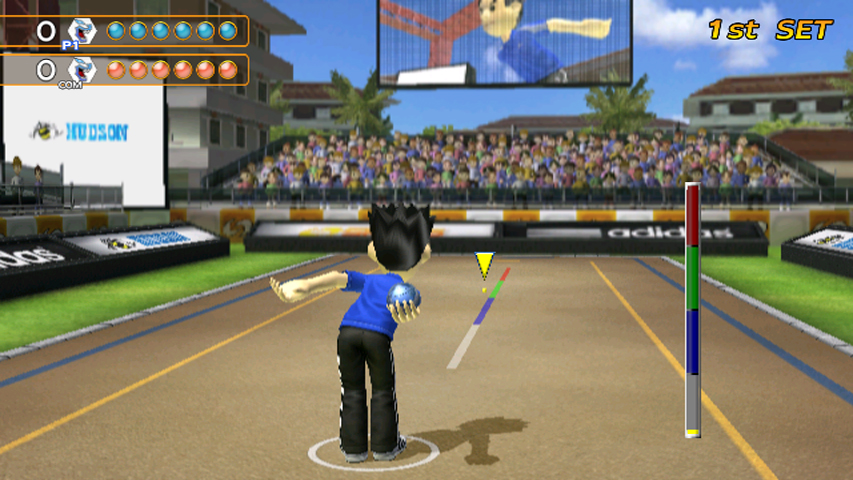A vibrant cartoon character, poised for action, is depicted ready to roll a blue ball, potentially playing bocce. With his hands bent backwards holding the ball, his black, spiky hair complements his ensemble of black pants and a blue shirt. The sun casts his shadow clearly on the ground. He is aiming to score points on a segmented graph colored gray, purple, green, and red, indicating distance or scoring zones. In the background, a blurred crowd watches intently, adding to the atmosphere of anticipation. The scene is set under a serene blue sky peppered with puffy clouds, bordered by palm trees and distant buildings. The character stands on a grassy track inside a distinct white circle, capturing the essence of a lively, outdoor athletic event.